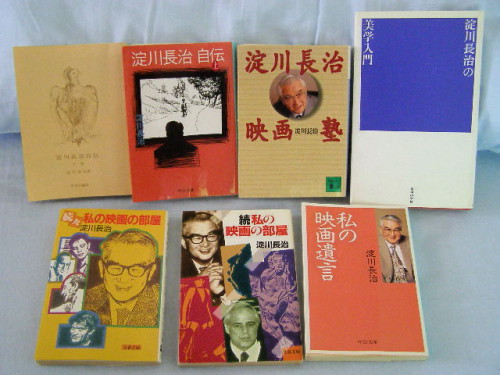This photograph showcases a collection of seven softcover booklets or pamphlets featuring what appears to be Chinese, Japanese, or Korean writing. The booklets are arranged in two rows on a light blue surface, possibly fabric. The front row consists of three booklets laid flat, while the back row has four booklets standing upright, leaning against the same light blue fabric backdrop.

Most of these pamphlets prominently display photographs or illustrations of an elderly man with whitish-gray hair and dark-rimmed glasses, likely a central figure or author, though his exact identity is unclear due to the unreadable script. These images vary in presentation but frequently reoccur across multiple covers, indicating a thematic or authorial connection.

The first booklet in the back row is beige with brown writing and a minimalist pencil sketch, while the second is red with a black and white photo resembling a TV screen. The third in this row is another beige booklet, featuring a red circle enclosing a man's photo, and the fourth booklet is primarily white, dominated by a blue square with white text.

In the front row, the first booklet is yellow with red letters and multiple images of individuals, dominated by a larger photo of the same elderly man. The middle booklet has a more complex front, featuring multiple men depicted in various colors with red and black text. The last booklet in this row is salmon-colored, with a prominent image of a man in the upper right-hand corner, adorned with white and black lettering.

The entire arrangement gives a cohesive yet varied visual impression, showcasing an array of potentially linked but distinct contents.